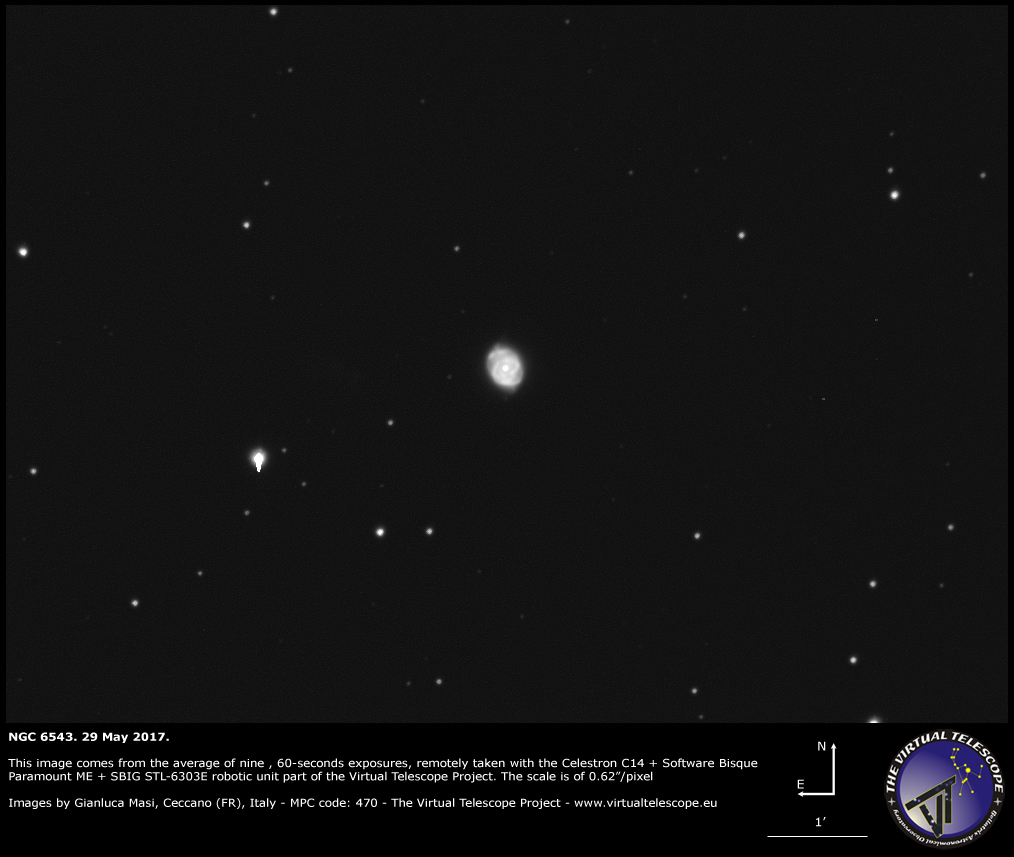In this black and white photograph of space, the vast darkness is punctuated by scattered white dots representing stars. Dominating the center of the image is a larger, spiral structure resembling a galaxy. At the bottom, a black horizontal strip contains detailed information in white text. The text reads: "NGC 6543, 29 May 2017," and provides technical details stating that the image results from the average of nine 60-second exposures remotely taken with the Celestron C14, B.I.S.C. Paramount ME plus SBIG STL-6303E robotic unit, all part of the Virtual Telescope project. The scale of the image is noted as 0.62 degrees per pixel. Also included are credits to Gianluca Massi from Cisano, FR, Italy, with an MPC code of 470, and a reference to the website www.virtualtelescope.eu. On the lower right of this strip is a circular logo featuring a purple sky and a telescope, inscribed with "The Virtual Telescope."